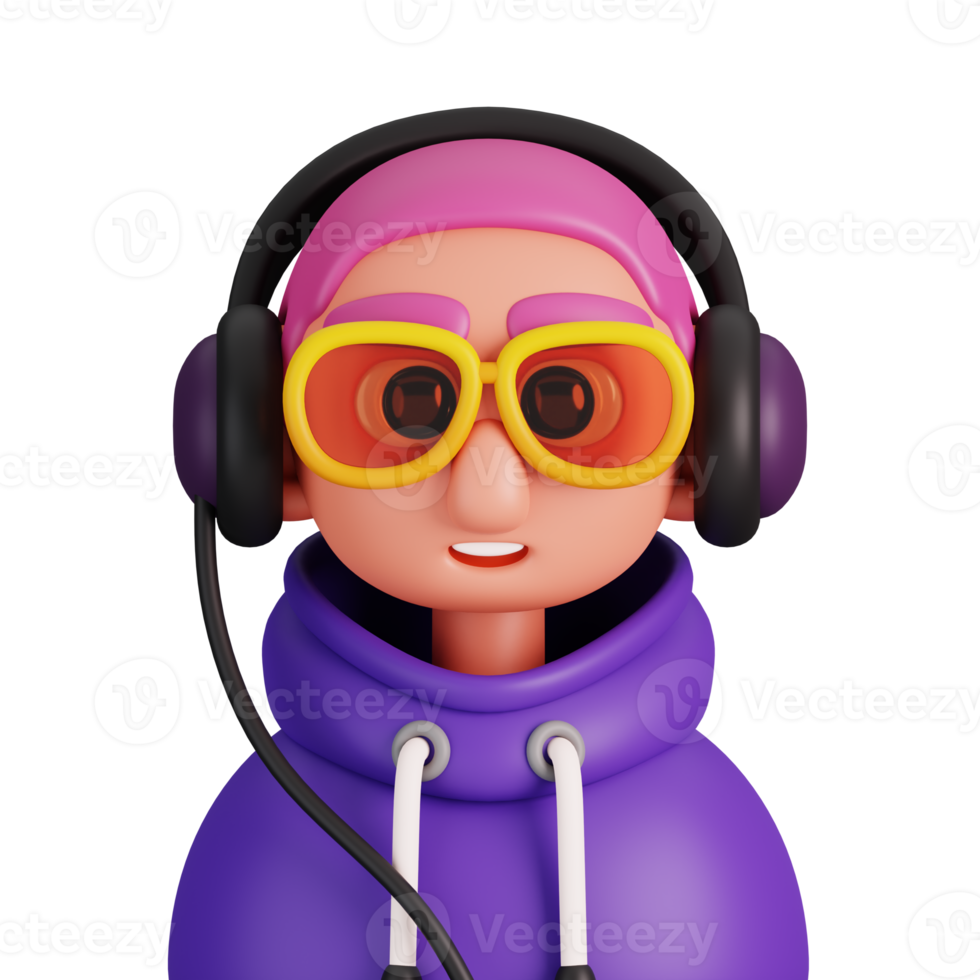The image depicts a computer-generated clay-like caricature in the form of a small toy figure. At the center of the image, set against a plain white background, the figure represents a young boy or character with a circular head and cylindrical neck, possibly intended to resemble an older lady, based on varying interpretations. The character is adorned with striking features: vivid pink hair and eyebrows, large yellow glasses with orange-tinted lenses, and oversized black headphones with purple details.

The figure dons a purple hoodie, complete with white drawstrings hanging down. The skin tone of the character is a beige, Caucasian color, albeit with a stylized, plastic-like texture. The face is marked by an elliptical, open mouth revealing white teeth, and large, round eyes with prominent circular irises. A noticeable black headphone cord extends down from one side of the headphones to the bottom of the image, adding to the realistic detail.

In the background, there's a subtle, yet distinct watermark displaying a "V" logo and the text "VEK TZ." This detailed and whimsical figure exudes a playful yet intricate design, combining elements of both a toy and a clay animation character.